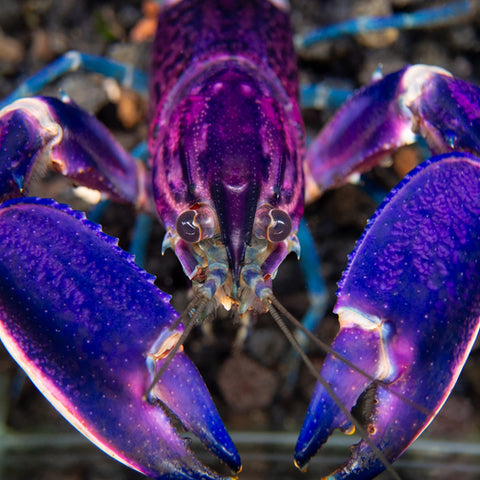This photograph captures a striking and unique clawed aquatic creature, resembling a lobster or perhaps a crawfish, primarily in vivid shades of purple and blue. The creature's entire body appears to be bathed in a fluorescent, almost UV-light-like glow that enhances its unusual coloration. The head and back of the creature showcase a mesmerizing pinkish-purple hue, while its large, moisture-dripping claws are a deep bluish-purple with hints of lavender. The critter's legs at the back are light blue, adding to the overall spectral palette. Prominent on its face are two sets of antennae-like whiskers and striped, hook-like features below its eyes. The eyes themselves seem directed towards the viewer. The background of the image is blurred, focusing all attention on this rare and vibrant specimen, presenting a breathtaking display of violet, lavender, and blue tones.